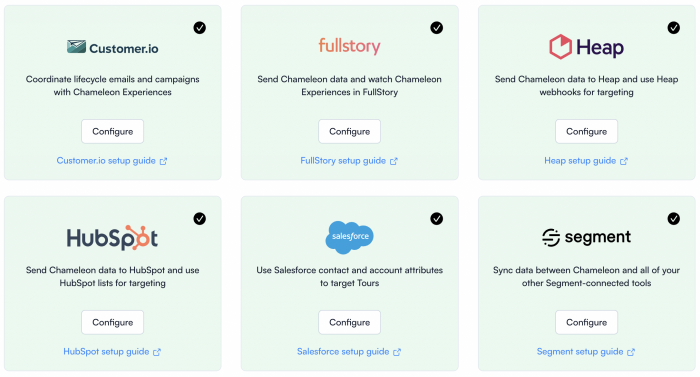The image features a grid of six boxes, arranged in a three-by-two layout. Each box has a light green background and contains distinct information along with a consistent interface element—a white button labeled "Configure" in black text.

**Top Row:**
1. **Customer.io**: The top-left box provides details about integrating Customer.io with Chameleon. It reads, "Coordinate lifecycle emails and campaigns with Chameleon experiences." Below the description is a blue link titled "Customer.io Setup Guide."
2. **FullStory**: The middle box in the top row discusses using FullStory with Chameleon. It states, "Send Chameleon-like data and watch Chameleon experiences in FullStory." A blue link below offers a "FullStory Setup Guide."
3. **Heap**: The top-right box covers integration with Heap, mentioning, "Send Chameleon-like data to Heap and use Heap webhooks for targeting." It also includes a blue link, "Heap Setup Guide."

**Bottom Row:**
1. **HubSpot**: The leftmost box in the second row is about integrating HubSpot with Chameleon. It says, "Send Chameleon-like data to HubSpot and use HubSpot lists for targeting." A blue link is provided as the "HubSpot Setup Guide."
2. **Salesforce**: The middle box in the bottom row focuses on Salesforce integration. It reads, "Use Salesforce contact and account attributes to target tours." Below it, there's a blue link titled "Salesforce Setup Guide."
3. **Segment**: The bottom-right box discusses using Segment with Chameleon. It states, "Sync data between Chameleon and all your other Segment data tools." The accompanying blue link is labeled "Segment Setup Guide."

Each box consistently presents a white "Configure" button to initiate the setup process.